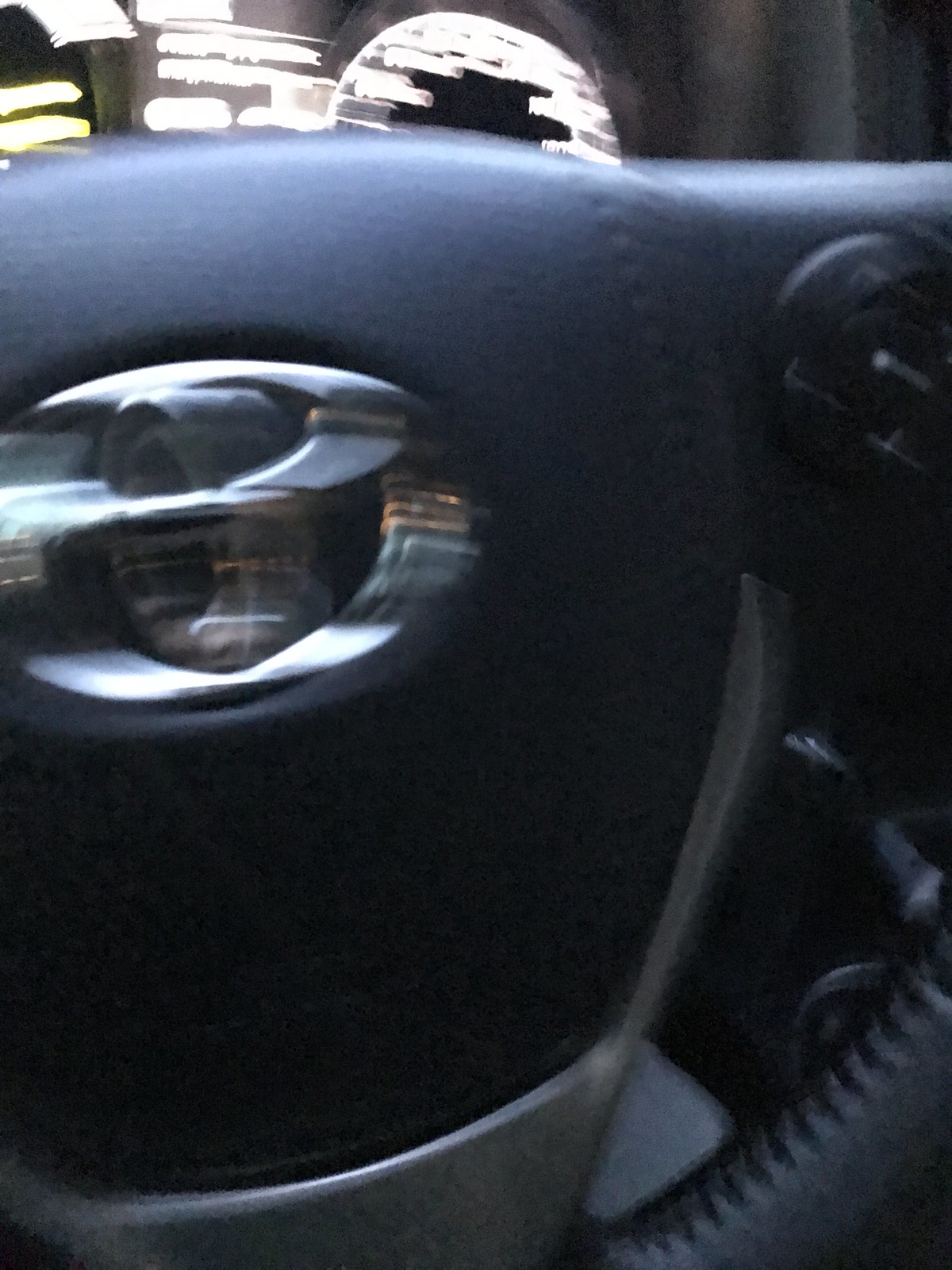This image is a blurry and somewhat distorted close-up of a car's steering wheel, predominantly dark gray in color. The photo is taken very close to the lower portion of the steering wheel, showing a leather-wrapped segment. A silver logo—potentially Toyota or Subaru—sits in the center, but it's too fuzzy to identify precisely. In the lower right corner of the image, a small black button with a silver stripe is visible, likely part of the car's control panel. The background features a mix of dim white and yellow dashboard lights, which include the odometer and other instrument readings, though these are also obscured by the blur. The image orientation is vertical, with some slight visibility out the window in the upper left corner. The shot includes elements that suggest either radio controls or additional steering wheel buttons on the right side.